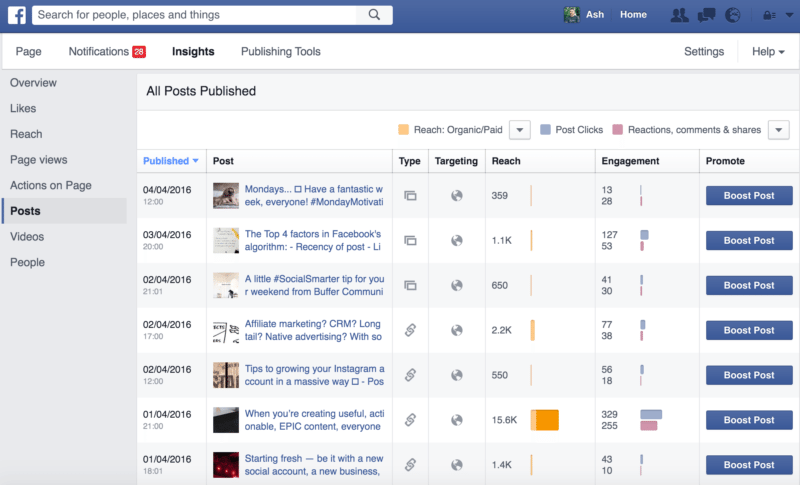A nostalgic glimpse into the early days of social media, this screenshot captures an old version of Facebook's web interface. Dominated by the signature blue banner, the top-left corner features the classic Facebook logo followed by a functional search bar to its right. Adjacent to the search bar, a row of categories distinctly labels 'Pages,' 'Notifications,' 'Insights,' and 'Publishing Tools,' providing an organized navigation experience.

Below, a section titled 'All Posts Published' introduces a series of posts displayed in list format. Each post is accompanied by various metrics, including engagement statistics, reach, targeting type, and a 'Promote' option, reflecting the analytical tools available to users. The streamlined design and straightforward layout evoke a sense of simplicity and a reminder of Facebook's evolving user interface over the years.